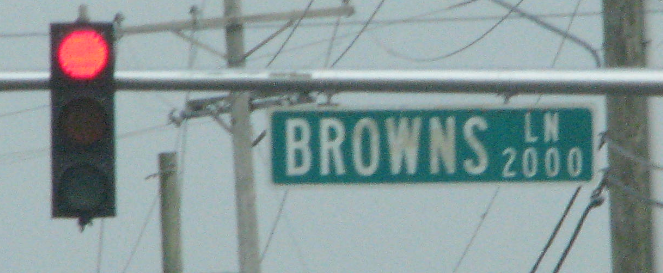The image depicts a red traffic light mounted on a metal pole, glowing brightly to signal vehicles to stop. Adjacent to the traffic light is a green street sign attached to the same pole, displaying the name "Browns Lane 2000" in white letters, indicating the street is named Browns Lane and its mile marker or address number begins at 2000. The background reveals numerous wooden utility poles, intricately networked with power lines that stretch across the scene. Above, a densely overcast sky looms, casting a subdued and gloomy ambiance over the street intersection.